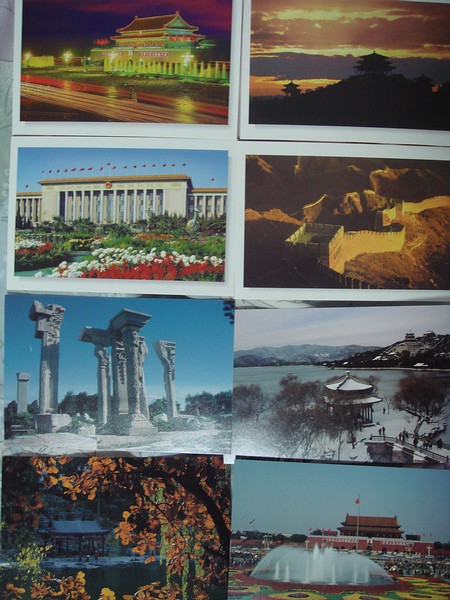This image showcases a collage of eight glossy postcards arranged in two columns of four. Each postcard captures a landmark or scene from around the world, though the majority seem to depict iconic sites in Asia. The top row features two postcards, one displaying an intricately layered Pagoda Temple and the other showing a similar style of Asian architecture, possibly during sunset and nighttime respectively. The second row includes the Great Wall of China on the right and a gray building surrounded by red flags and green, red, and white flowers on the left. 

On the third row, the right postcard depicts a snow-covered building with barren trees, while the left postcard features ancient stone pillars reminiscent of ruins in Athens. The bottom row includes a majestic fountain next to a reddish building on the right, and a serene scene of green and brown leaves with a bench in the middle on the left. Notably, the top four cards are adhered to a larger white sheet, while the bottom four are standalone. The photo captures slight reflections on the luminous photo paper, hinting at its glossy finish, and shows that the postcards are not perfectly centered within the frame.